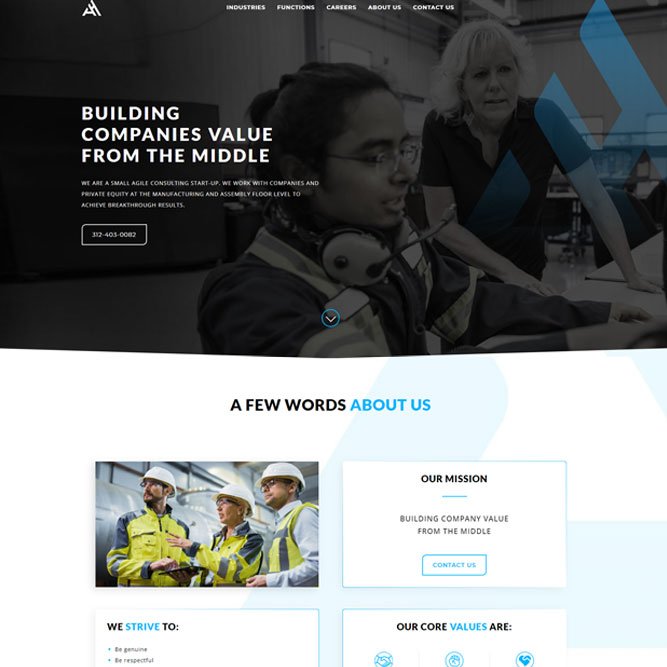In the upper portion of the screenshot, there's an image featuring two women in a grayscale, photograph-style picture. The first woman, seated, has dark hair tied back and is wearing glasses. She appears to be speaking into a microphone, her headphones in place, possibly engaging in a discussion or broadcast. Beside her, either seated or standing, is an older woman with short blonde hair, wearing a black t-shirt, her hands steadying herself on a desk. The background suggests an office setting. On the left side of this image, there's text reading "BUILDING COMPANY'S VALUE FROM THE MIDDLE" in all caps white letters. At the top-left corner of this portion, there's a logo resembling the letter "A" followed by smaller, white capitalized text stating "INDUSTRIES AND FUNCTIONS CAREERS ABOUT US CONTACT US." Below the main text, there's a section with three lines and a code or number in a box outlined in white.

The lower portion of the screenshot contains a second image with some text elements. At the top, in all-caps black letters, are a few words followed by "ABOUT US" in blue, also in all caps. To the left, there's an image of three individuals wearing helmets and safety gear, predominantly in dark yellow, gray, and white hues. They appear to be in a laboratory setting. The group consists of a woman in the middle and two men to her sides, all gazing to the left. One man holds a piece of paper, and the woman is pointing at something within their view. Below this image, in black and blue text, it reads: "WE STRIVE TO: BE GENUINE AND BE RESPECTFUL," with two blue dots following the phrase. To the right, within a box, are the words "OUR MISSION" in black, all caps, underlined in blue. The text beneath states, "BUILDING COMPANY VALUE FROM THE MIDDLE," and includes a "CONTACT US" button outlined in blue with blue text. Below that, "OUR CORE VALUES" are displayed in black and blue all-caps, with the acronym "R-A-R-E" highlighted in black type. Finally, at the bottom are three icons; although unclear, the one to the far right resembles a heart with a line through it.